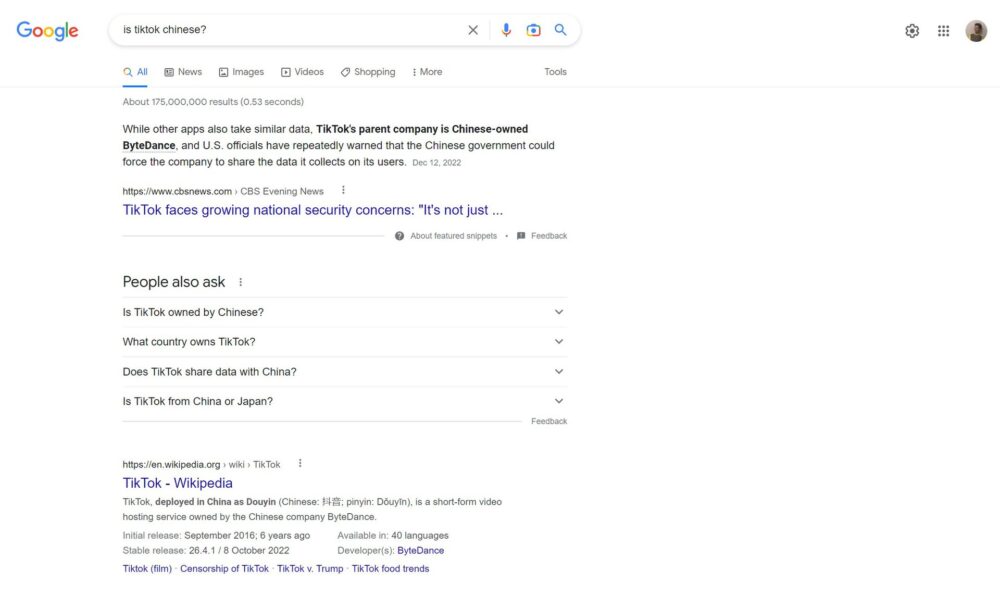The image captures a horizontally oriented, high-resolution screenshot of a Google search page on either a tablet or a desktop. The interface is in its classic white theme, featuring the distinctive, multicolored Google logo in the top-left corner. In the search bar, the user has typed the query, "Is TikTok Chinese?" The familiar icons for voice search (microphone), image search (camera), and the magnifying glass for initiating the search are clearly visible next to the search box.

Below the search bar, the default search categories are displayed: "All" (highlighted in blue), "News," "Images," "Videos," "Shopping," and "More," with "Tools" positioned to the right after a small gap. The top search result, sourced from CBS News and dated December 12, 2022, briefly states: "While other apps also take similar data, TikTok's parent company is Chinese-owned ByteDance, and US officials have repeatedly warned that the Chinese government could force the company to share the data it collects on its users."

Further down, the "People also ask" section provides additional queries related to the main search, such as "Is TikTok owned by Chinese?" "What country owns TikTok?" "Is TikTok shared data with China?" and "Is TikTok from China or Japan?" At the bottom of the visible search results, there's a link to TikTok's Wikipedia page, containing general information about the app, including its initial release and most recent stable release date.